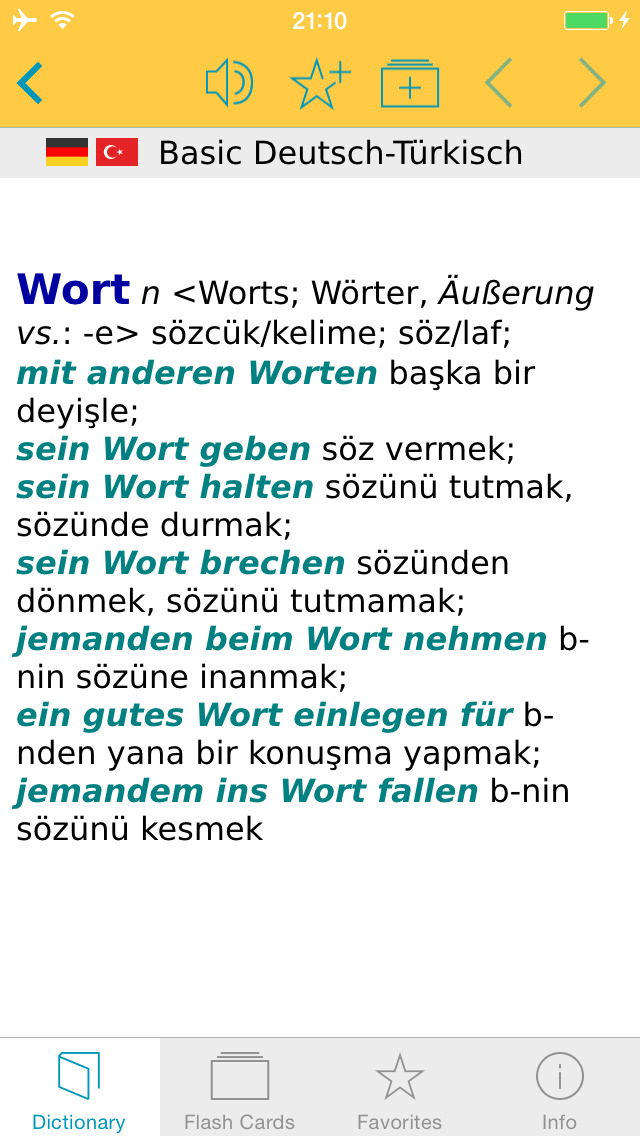The image depicts a mobile app screen resembling a dictionary webpage, written in a mix of German and Turkish. At the top of the screen, there is a yellow header containing various symbols including an audio speaker, a star with a plus sign, a folder with a plus sign, and navigation arrows pointing left and right. Additionally, the top left corner displays an airplane mode icon with a Wi-Fi symbol next to it, and the time is shown as 21:10 in the middle. The battery icon on the top right indicates a full charge.

Below the header, there are flags of Germany and Turkey alongside the text "Basic Dutch/Turkish" written in black, suggesting a translation app from Dutch to Turkish or vice versa. The main body of the screen includes the word "Wort" in blue, signifying a German noun, along with its definitions and translations. The German text is in a light blue-green color and the Turkish text is in black. Some of the German definitions listed are "wart geben, sos vermak" and "wart halten, sozunu tutmak."

At the bottom of the screen is a horizontal rectangle with tabs indicating dictionary functions: "Dictionary" highlighted in blue with a book icon, followed by "Flashcards" with stacked rectangles, "Favorites" with a star, and "Info" with a circular icon containing an 'i'. The background of this section is light gray, complementing the functional imagery of the app.

The design incorporates various colors, predominantly blue, yellow, black, and a blend of light blue-green and lavender hues. The overall layout is vertical, typical of a mobile dictionary app geared towards bilingual translation and definitions.